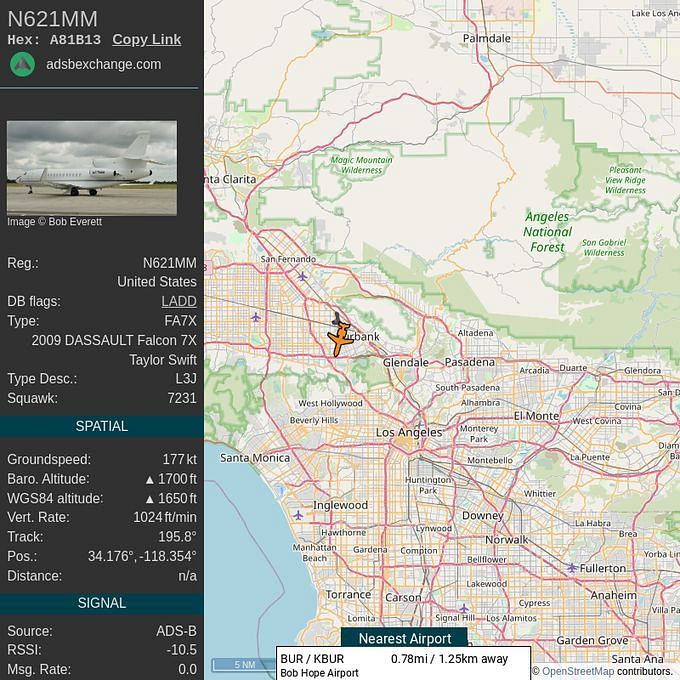This image displays a flight tracking interface featuring detailed real-time information about a specific aircraft with the registration number N621MM, owned by Taylor Swift. Captured by Bob Everett, this aircraft is a Dassault Falcon 7X, with the specific type identifier FA-7X-2009DAF-7X and type description L3J. The hex code for this aircraft is A8-1B13, and it is flagged with DB for LADD (Limiting Aircraft Data Displayed).

Key flight parameters include a squawk code of 7231, a ground speed of 177 knots, a barometric altitude of 1,700 feet, and a WGS 84 altitude of 1,650 feet. The aircraft's vertical climb rate is noted at 1,024 feet per minute, and it is on a course of 195.8 degrees. Its geographical coordinates are 34.176° North and 118.354° West, placing it over Burbank, Los Angeles. The nearest airport is Burbank or Bob Hope Airport, located just 0.7 miles away.

The data is sourced from ADS-B (Automatic Dependent Surveillance-Broadcast) with an RSSI (Received Signal Strength Indicator) value of -10.5. The interface includes a map panel showing the aircraft's precise location, with a detailed account of its flight path, altitude, and speed.

This comprehensive tracking system offers an in-depth view of Taylor Swift's privately owned aircraft, ensuring real-time monitoring of its movements and proximity to critical locations.